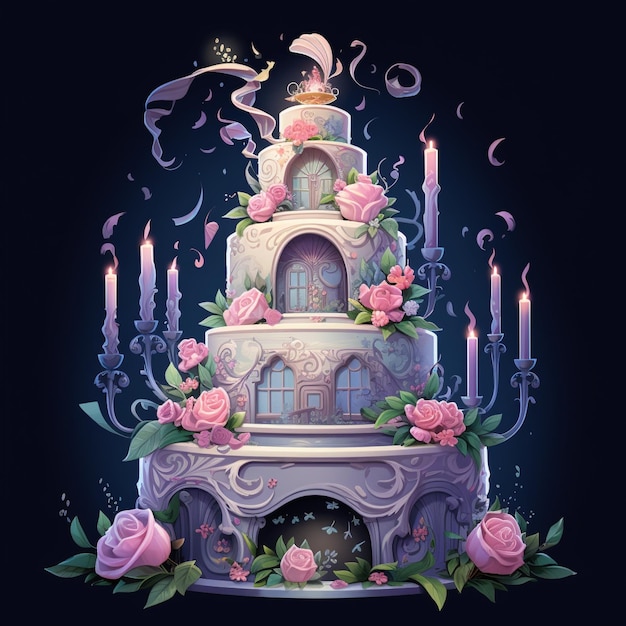This digital artwork, likely AI-generated, features an elaborate five-layer cake set against a dark blue background that gradually lightens towards the cake. The cake is reminiscent of a castle or building, adorned with various intricate details. It has pink roses scattered around and an archway at the bottom, partially hidden behind one of the roses. The second, third, and fourth layers incorporate embedded windows, enhancing the architectural feel. The second tier has unevenly sized candles on either side, with three lit candles grouped together in candleabras. The third tier also features a candleabra on each side. The frosting on the cake has sophisticated curved designs, contributing to its ornate appearance. At the top, a small golden bowl with flames emerging from it crowns the cake, adding a final touch of grandeur. Additionally, there are subtle visual effects such as curves in the frosting that appear to float mid-air, resembling snowflakes or cream, further enhancing the whimsical aesthetic of the cake.